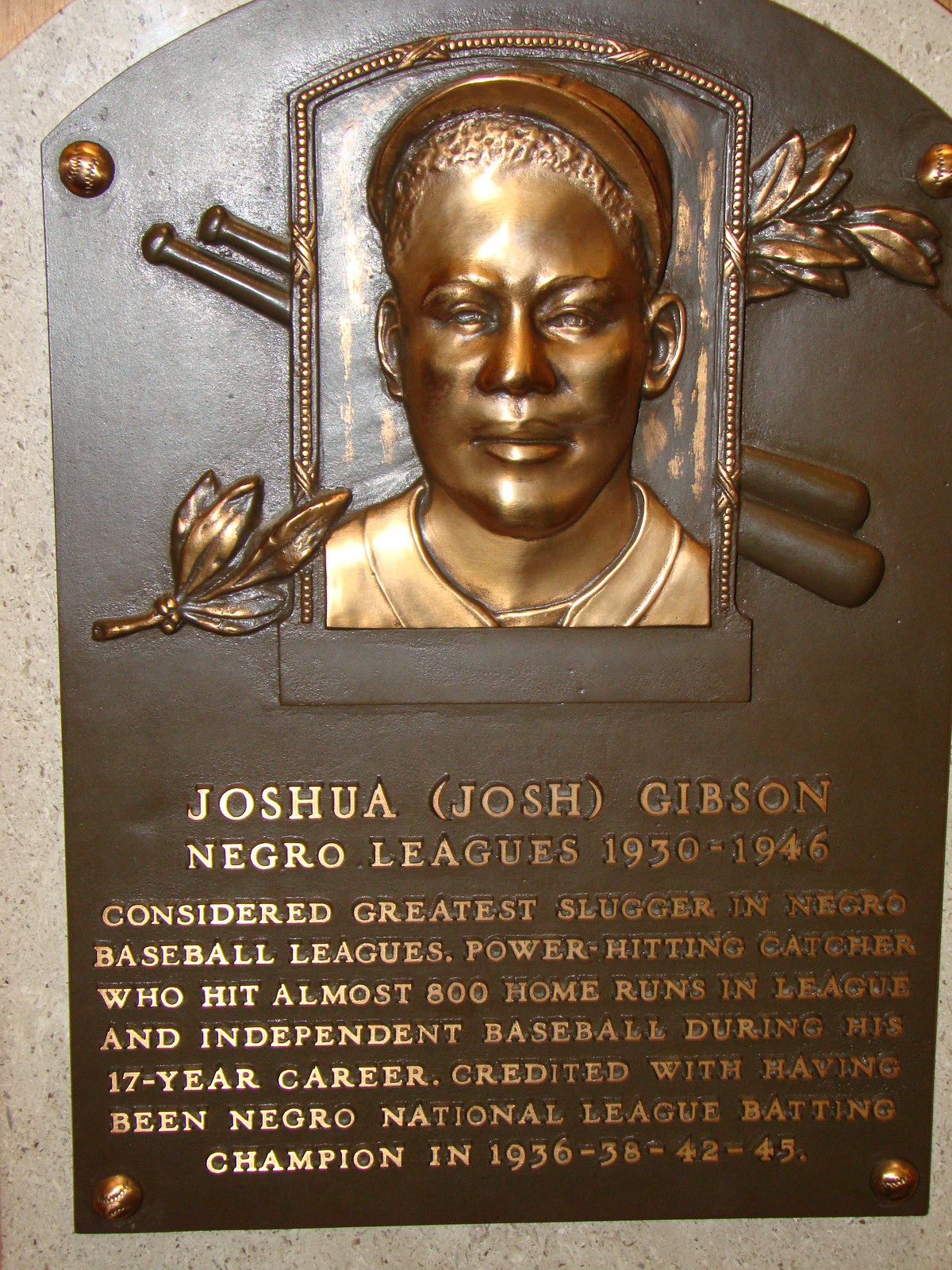This informational plaque honors Joshua "Josh" Gibson, one of the greatest sluggers in baseball history, renowned for his extraordinary achievements in the Negro Leagues from 1930 to 1946. The plaque, cast in bronze and bordered in granite, features a headstone shape with a relief image of Gibson's head and upper shoulders in a baseball uniform, flanked by laurel leaves and crossed baseball bats. Inscribed in uppercase font are his name and career details, including his tenure as a catcher and slugger in the Negro Leagues. Gibson, who hit nearly 800 home runs over a 17-year career, was the Negro National League batting champion in 1936, 1938, 1942, and 1945. This monument stands as a testament to Gibson's exceptional legacy and the rich history of segregated baseball.